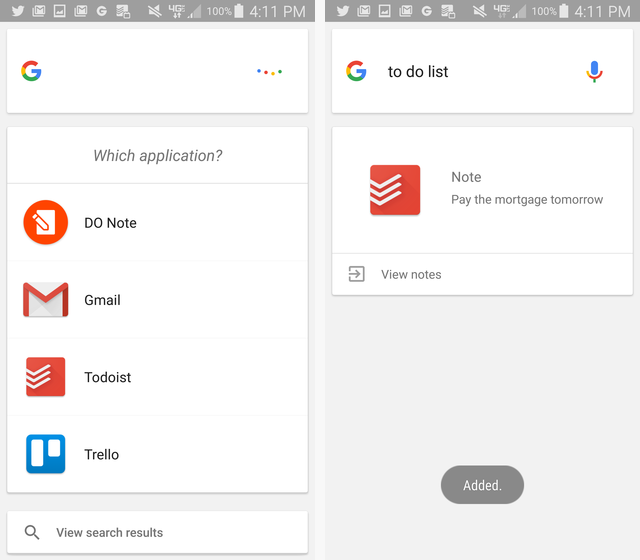This image features two side-by-side screenshots of a smartphone, displaying identical notification bars at the top. The notifications include a Twitter alert, an email notification, an alert from Photos, another email notification, and a Google app alert. Additional icons present are for Box, a muted sound icon, a 4G network indicator, a symbol for signal bars, a 100% battery level, and the time showing 4:11 p.m.

In the first screenshot, there is a Google search prompt at the top, reading "Which application?" underlined by a white box. Below are four selectable options: "Do Note," symbolized by a red circle with a pen and paper icon; "Gmail," depicted with an envelope icon; "Todoist," represented by a red box with white lines; and "Trello," shown as a blue box with two different-sized rectangles. At the bottom, an option to view search results is present.

The second screenshot mirrors the notification bar of the first. It also features a Google search prompt but lists "Todoist" beside a microphone icon, followed by a note that reads, "Pay the mortgage tomorrow."